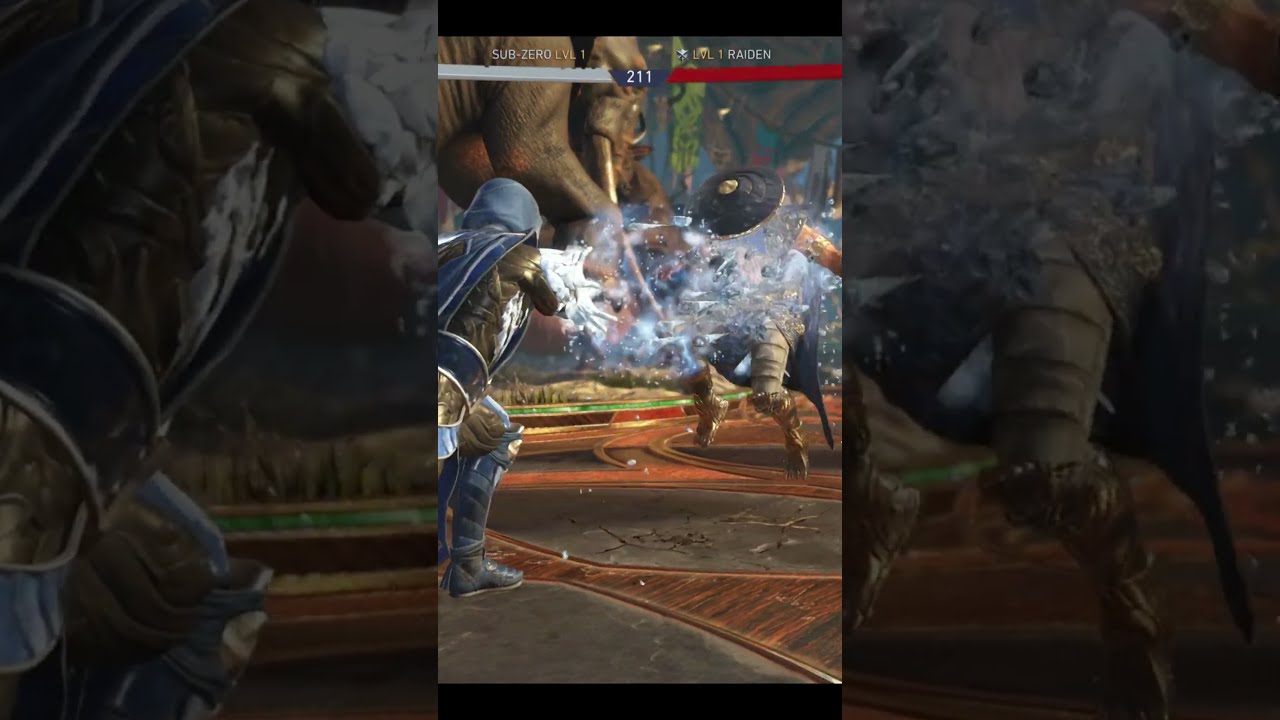This image is a detailed screenshot from a video game showing a dynamic battle scene. In the foreground, you see a fierce confrontation between two characters: one is a warrior clad in gold armor with a blue cape and black shoes, and he appears to be hurling an object at his opponent. The opponent, who has black headgear and orange sleeves, is airborne and barefoot, partially obscured by the thrown object. The scene is set on a street-like surface, characterized by gray concrete interspersed with red areas and possibly wood or granite inlays.

Dominating the backdrop, a giant dinosaur-like creature with tusks and a see-through body featuring blue and brown colors looms over the fighters. To add further depth, a variety of flags hang in the distance, and patches of green can be seen beyond the immediate battle area. A white stripe bisects the screen, with blue and red sections displaying scores or levels, indicating Sub-Zero at Level 1 and Level 1 Raiden, respectively. The overall image is framed by larger, grayed-out versions of the central scene, providing a dramatic and immersive border.